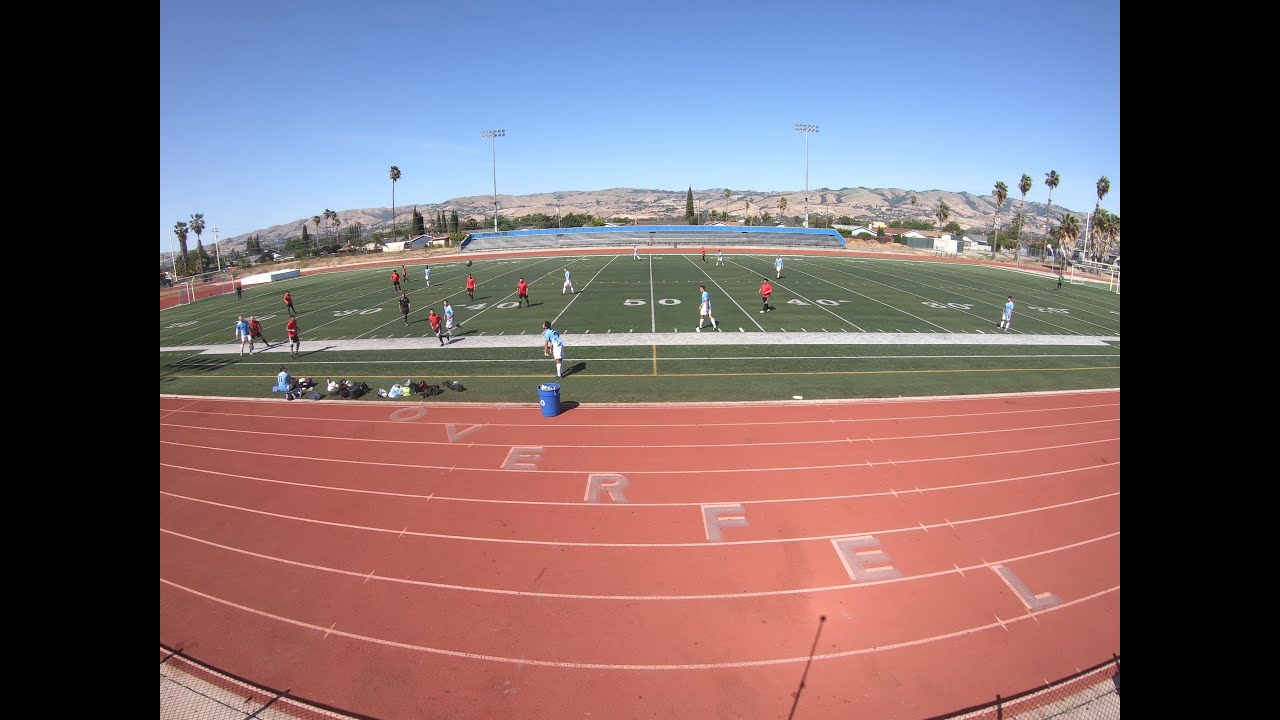The image captures a vibrant scene on an outdoor high school football field surrounded by a red track with each lane marked by a single letter spelling out O-V-E-R-F-E-L. Centered on the lane nearest the lush green grass of the football field is a blue trash can. The field is meticulously maintained, with short, vivid green grass and white lines and numbers designating various sections. Players are engaged in a dynamic soccer match, with one team donning orange shirts and black pants, while the other team sports blue shirts and white pants. Spectators may be observing from the bleachers, given the photo perspective. The weather appears sunny with a clear blue sky, adding a bright backdrop to the scene. In the distance, dusty hills and palm trees flank the field, suggesting a warm, desert-like environment, possibly Arizona. The lively atmosphere points to an afternoon game, with kids actively playing and the surroundings bathed in sunlight.